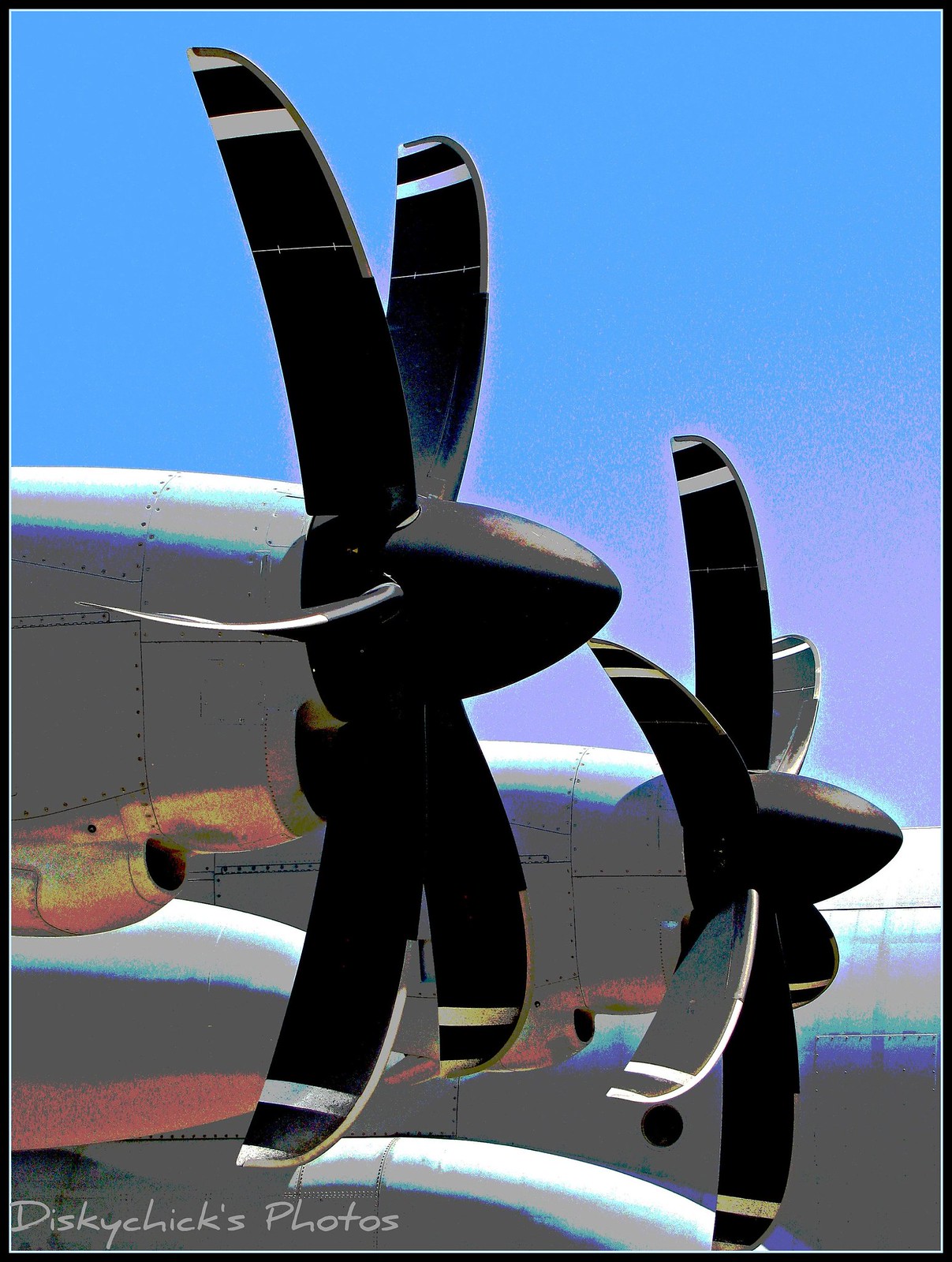The image depicts a meticulously painted scene at an airport environment featuring the iconic elements of a silver, vintage airplane characterized by its prominent rivets. The primary focus is on the airplane's stationary propellers. There are two visible propellers, each with a distinctive curved design and consisting of six blades, all painted black with white tips. The blades exhibit two silver stripes at their tips. The background of the painting gradates from a serene baby blue sky at the top to purple hues towards the center, finally transitioning to white near the horizon, suggesting early dawn or dusk. The lower section portrays a gray runway, providing a grounded perspective. The signature "Disky Chicks Photos" is visibly inscribed in white at the bottom left corner, indicating the artist’s identity. The overall texture and color highlight suggest a combination of traditional painting techniques with possible digital enhancements, adding to the vividness and depth of the scene. The use of contrasting colors, such as the subtle introductions of orange and red on the airplane fuselage, adds a surreal, almost nostalgic feel to the image.